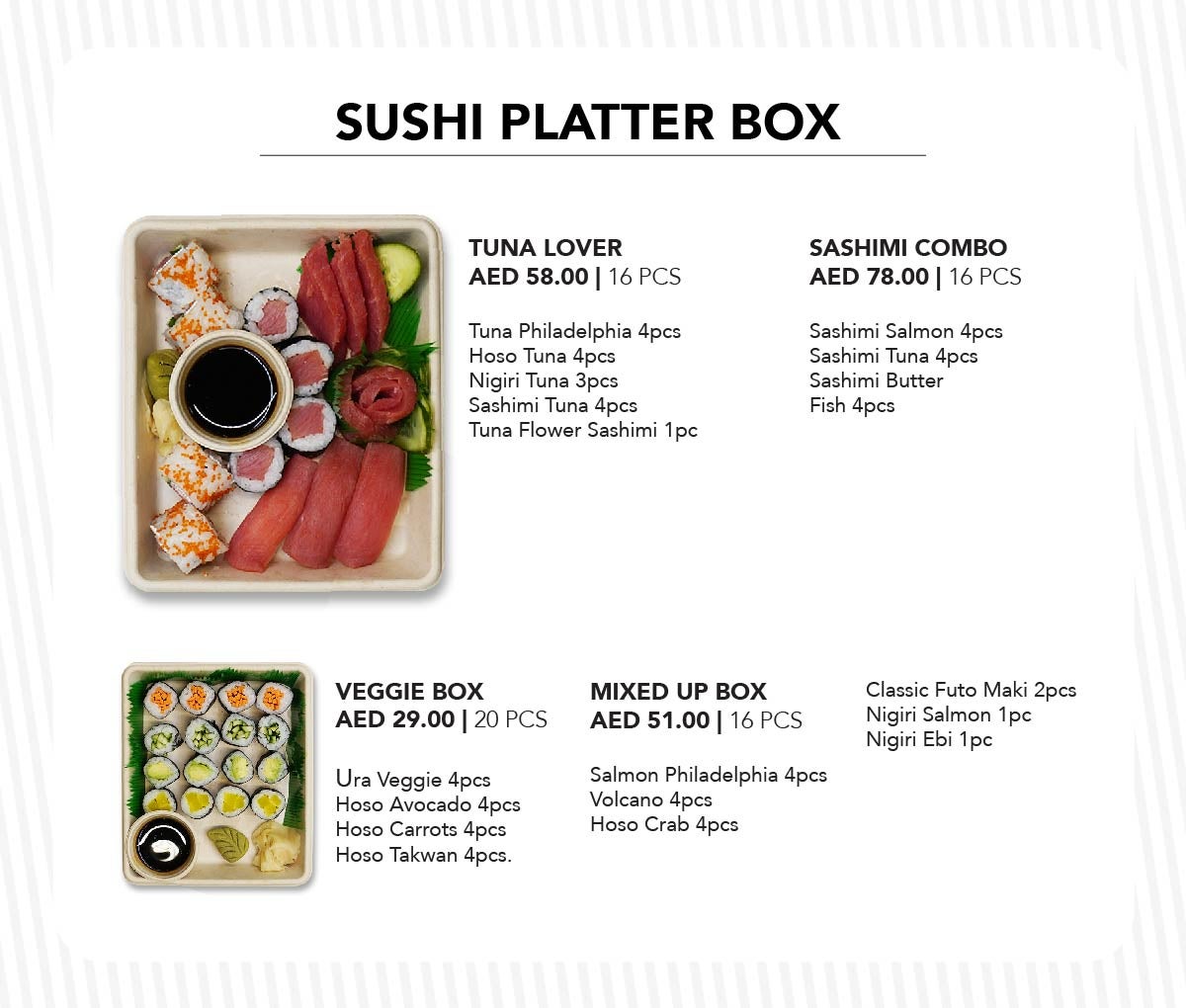This image showcases a detailed menu for sushi platter boxes, presented inside a white rounded rectangle against a background of gray diagonal lines. The top of the menu displays "SUSHI PLATTER BOX" in bold black letters. 

On the left side, there's a tan tray with various types of sushi, accompanied by a small ramekin of brown liquid, likely soy sauce. Adjacent to this tray, in bold black font, it says "TUNA LOVER," priced at AED 58.00 for 16 pieces. The tray includes detailed labels for each sushi type: 4 pieces of Tuna Philadelphia, 4 pieces of Hoso Tuna, 3 pieces of Nigiri Tuna, 4 pieces of Sashimi Tuna, and 1 piece of Tuna Flower Sashimi.

To the right, there is another column with "SASHIMI COMBO" priced at AED 78.00 for 16 pieces. This combo includes 4 pieces each of Sashimi Salmon, Sashimi Tuna, Sashimi Butterfish, and Sashimi.

Below the Tuna Lover section, there is another tray labeled "VEGGIE BOX" priced at AED 29.00 for 20 pieces. This box features 4 pieces each of Yura Veggie, Hoso Avocado, Hoso Carrots, and Hoso Takuan.

Next to the Veggie Box is the "MIXED UP BOX" priced at AED 51.00 for 16 pieces, listing 4 pieces of Salmon Philadelphia, 4 pieces of Volcano, and 4 pieces of Hoso Crab. Additionally, it includes Classic Futo Maki (2 pieces), Nigiri Salmon (1 piece), and Nigiri Ebi (1 piece).

Overall, this menu offers a variety of sushi boxes, catering to different preferences with precise descriptions and vibrant images of the offerings.